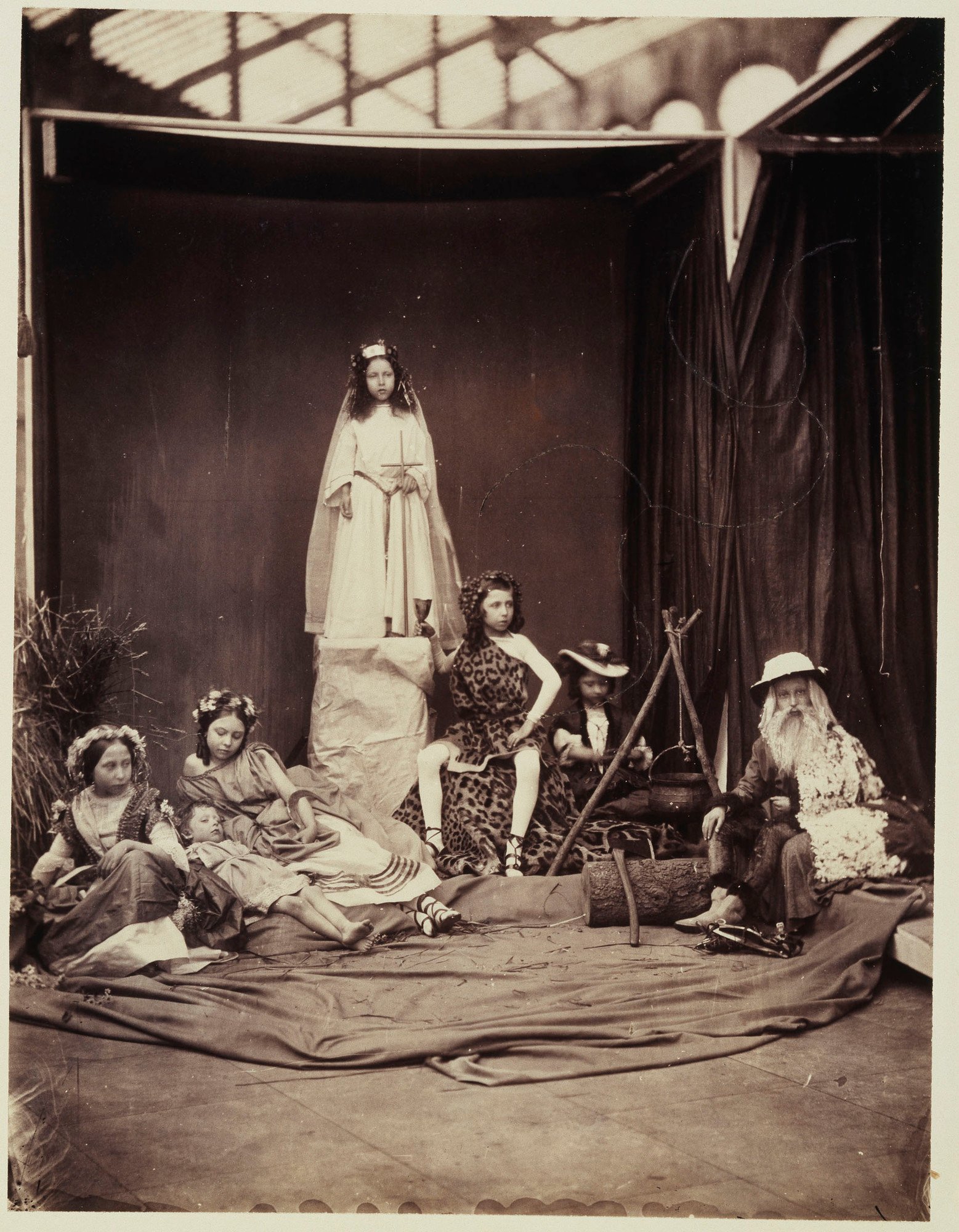This black-and-white photograph, which appears to be a picture of an older photo, captures seven children meticulously posed on a stage that resembles a primitive set. They are dressed in various costumes, suggestive of a possible historical or biblical scene. Each detail is rich in period-specific attire: the boy on the right wears a straw hat, a long fake beard, and white hair, exuding an elder's presence. In the center, a girl in a white dress stands elevated on a pedestal, crowned and clutching either a cross or a sword, her head draped with a shawl. At her feet sits another child in a leopard-print dress, holding a cup, evoking a primitive or regal air. Surrounding them are other children in white robes, two of whom recline adorned with flower hats, and an infant lies among them, possibly indicating a nativity scene. The backdrop is dark with heavy curtains, and props like a primitive campfire with a pot hanging from a stick triangle arrangement, enhance the scene's depth, transporting the viewer to a seemingly ancient tableau reminiscent of Bethlehem.